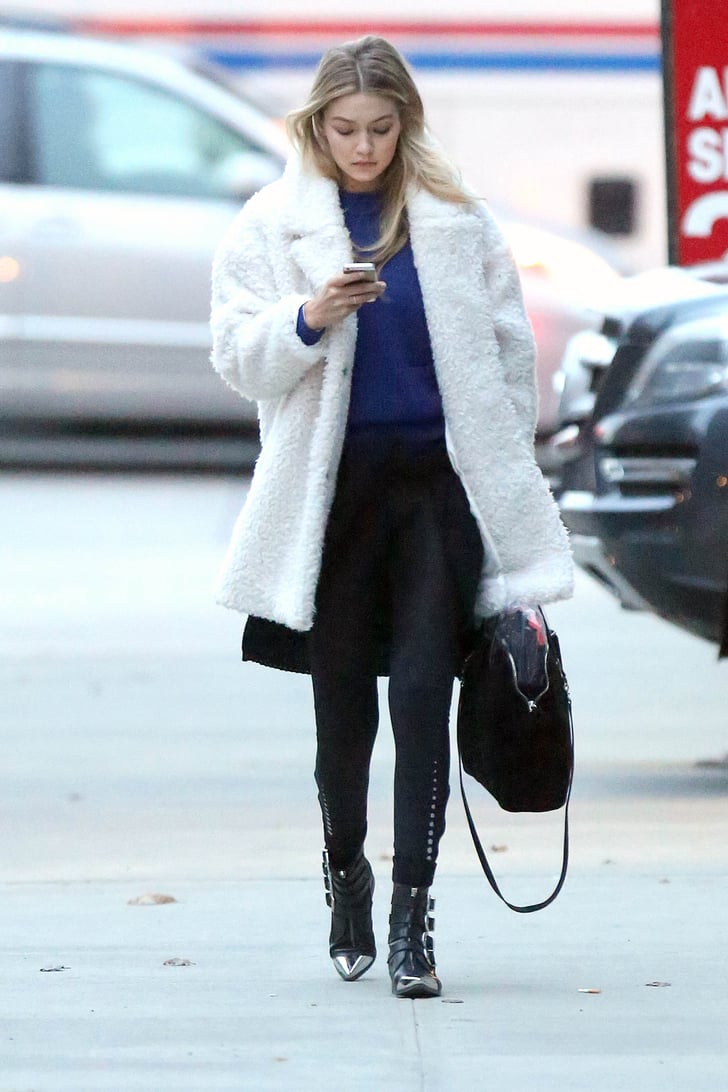In this color photo, a young woman in her early 20s, with mid-shoulder length blonde hair parted in the middle, is walking along a street while looking down at her phone with a serious expression. She's dressed in a white fuzzy coat over a navy blue top, paired with black pants or a black skirt and tights. Her ensemble is completed with black ankle boots featuring silver toes and buckles. She carries a large black handbag in her right hand, which has a strap that can be slung over her shoulder or held by shorter handles. The background includes a few muted, blurred cars, suggesting she might be walking through a parking lot or near a sidewalk, possibly outside a post office, given the out-of-focus building with a red and white stripe behind her. The scene appears to be set during the daytime.